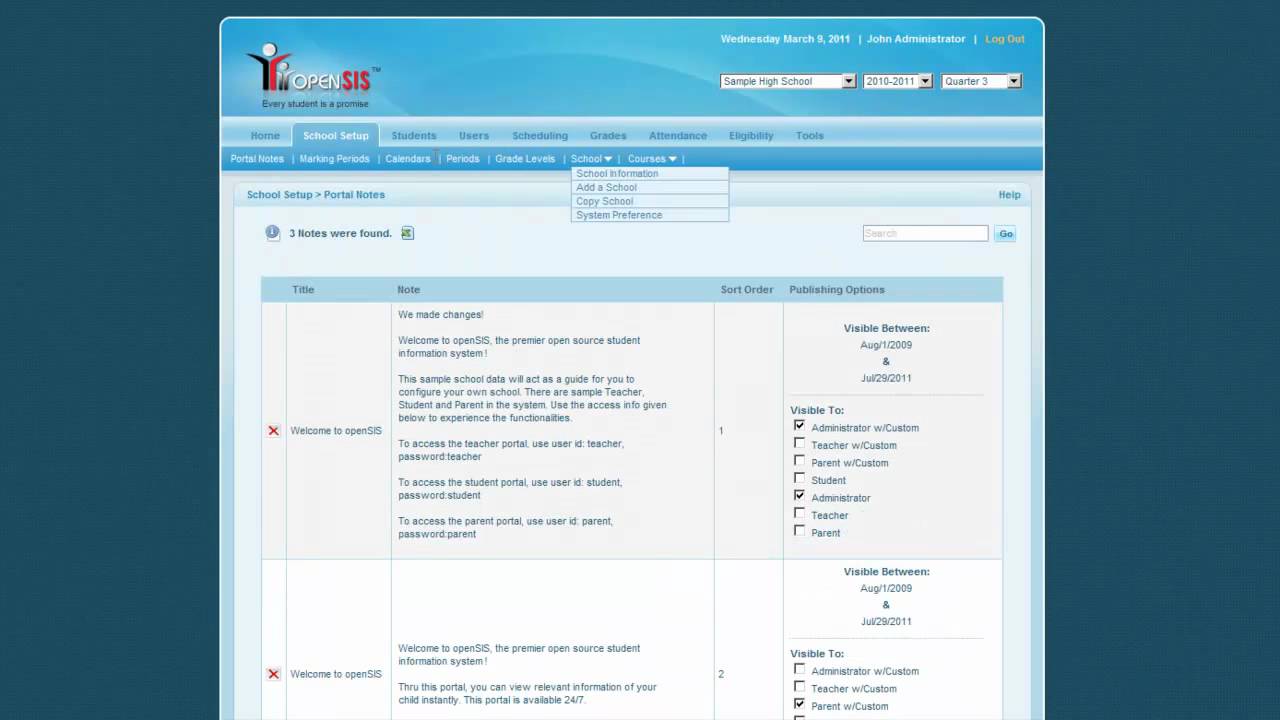The image depicts a webpage from a platform called "OpenSIS." The text on the page is relatively small, and a specific phrase suggests that "Every Student is a Promise." The navigation bar at the top of the page includes several tabs labeled: Home, School Setup, Students, Users, Scheduling, Grades, Attendance, and Eligibility Tools. The current view displays the "School Setup" section, which expands into more subsections such as Portal, Waiting Periods, and Calendars. The Portal Notes subsection is highlighted, listing items like "Welcome to OpenSIS" and offering general information about the portal. The site design appears somewhat basic with a nostalgic feel, featuring a predominantly white and light gray background, accentuated by varying shades of blue throughout.